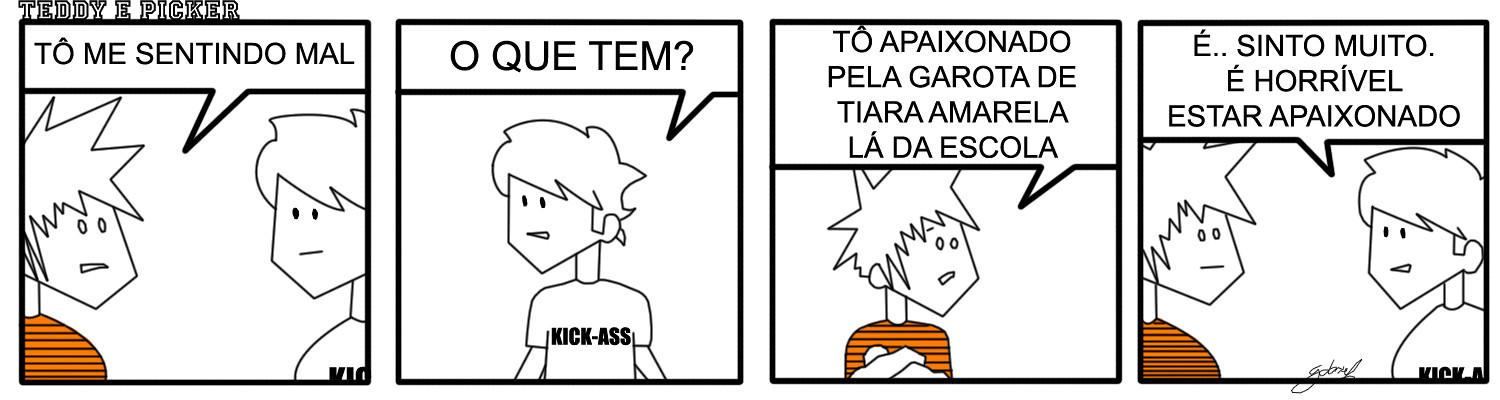The comic strip titled "Teddy E. Picker" is presented in four panels and appears to be in Spanish. 

1. **Panel 1**: In the top left corner of the comic, the text reads "Teddy E. Picker". The first panel features two characters: one with spiky hair and an orange shirt, who is speaking to another character rendered entirely in black and white. The character in the orange shirt is saying, "Tomy Centendo Mall."

2. **Panel 2**: The scene shifts to just the black and white character, who seems to be standing alone, appearing contemplative or perhaps waiting for a response.

3. **Panel 3**: The focus returns to the character in the orange shirt. This panel shows him alone, making a response, although the exact nature of his dialogue is not clear.

4. **Panel 4**: Both characters reappear, continuing their conversation. The black and white character responds back to the boy in the orange shirt, with an expression indicating engagement in the dialogue.

Although the specific dialogue in the final two panels is not provided, the comic strip evidently captures an interaction between these two distinct characters in a style reminiscent of traditional comic artistry.